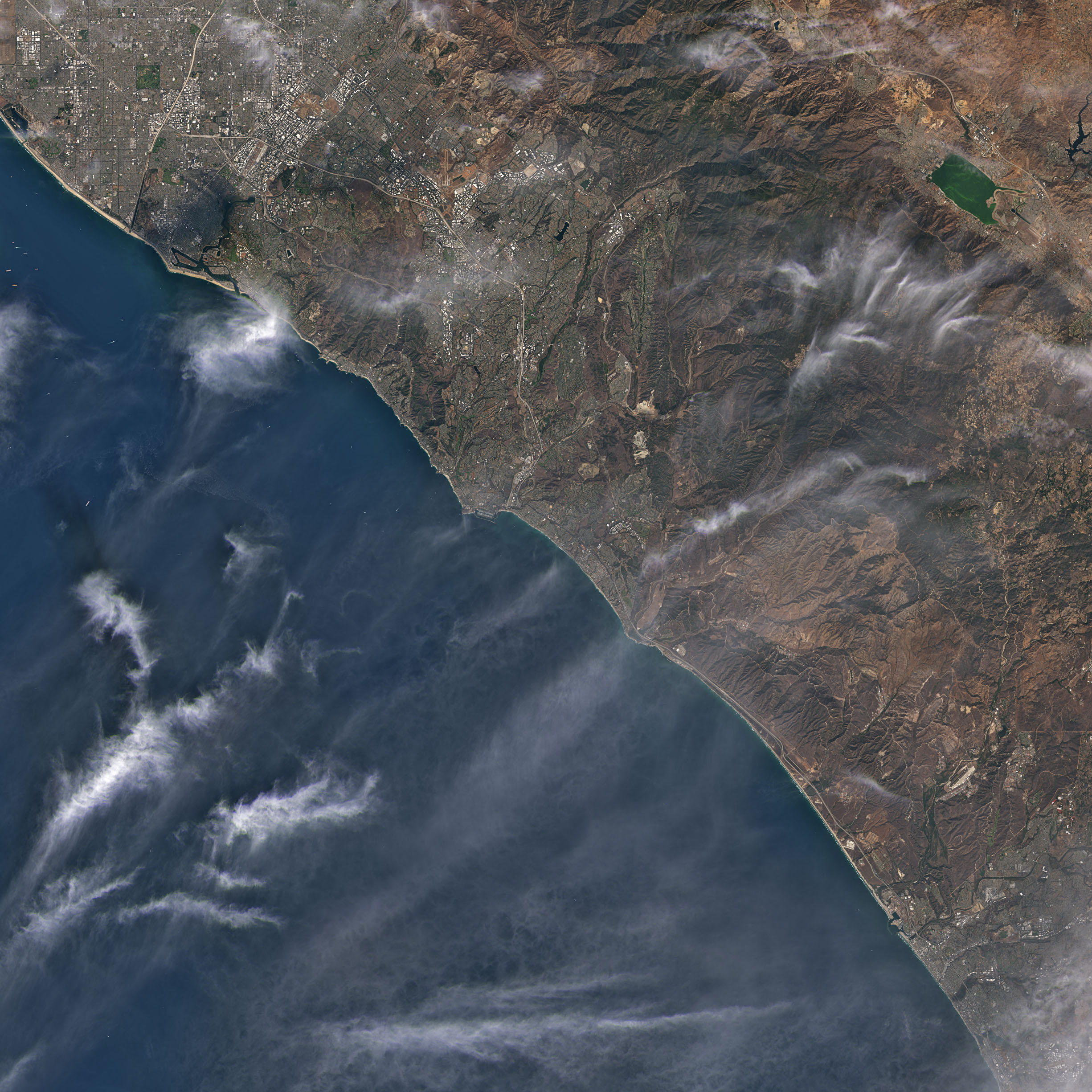This aerial or satellite photograph captures an expansive view of a coastline, likely in the western United States, including California or Mexico. The image is characterized by the striking contrast between the deep blue ocean waters on the left and the rugged, tan and rocky mountainous regions inland. Wispy white clouds are visible, scattered above the scene. The landscape showcases numerous valleys converging toward the sea, reflecting a rich topography of both geology and urban development.

In the top right corner, a green lake distinctively stands out amidst the landscape, suggesting a break in the otherwise arid and rocky terrain. The upper left portion of the image features city areas and sprawling suburbs marked by a noticeable crosshatch of roads, dotted with white building tops and roofs. Major roads are discernible, interlinking the cities and suburbs with the more mountainous areas inland.

Further detailed examination reveals various shades of brown, green, tan, and white along the coast, as well as some breaks and cracks in the rocky regions, particularly lighter gray rocks in the left and bottom corners. The coastline runs diagonally from the top left to the bottom right, suggesting a diverse environment with cliffs, potential towns, and more secluded dwellings.

Overall, this photograph, taken from several thousand feet above, presents a detailed visual narration of a dynamic and complex coastal region, with natural and human-made elements intricately woven into the landscape beneath a canopy of gentle clouds.